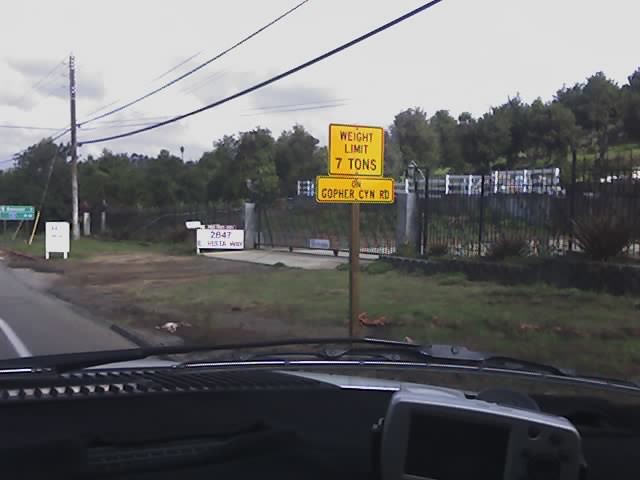The image captures a dashboard view of a fenced-off area, likely associated with a business, situated on the right side of a road. Prominently displayed in the center is a green road sign that reads "Weight Limit 7 Tons." To the right, amidst patches of green grass, there's a sign displaying numbers: "262847." The background reveals a bit of green landscape, and the sky above is dotted with fluffy white clouds. Overhead, power lines stretch across the top portion of the image, further enhancing the scene's depth and realism.